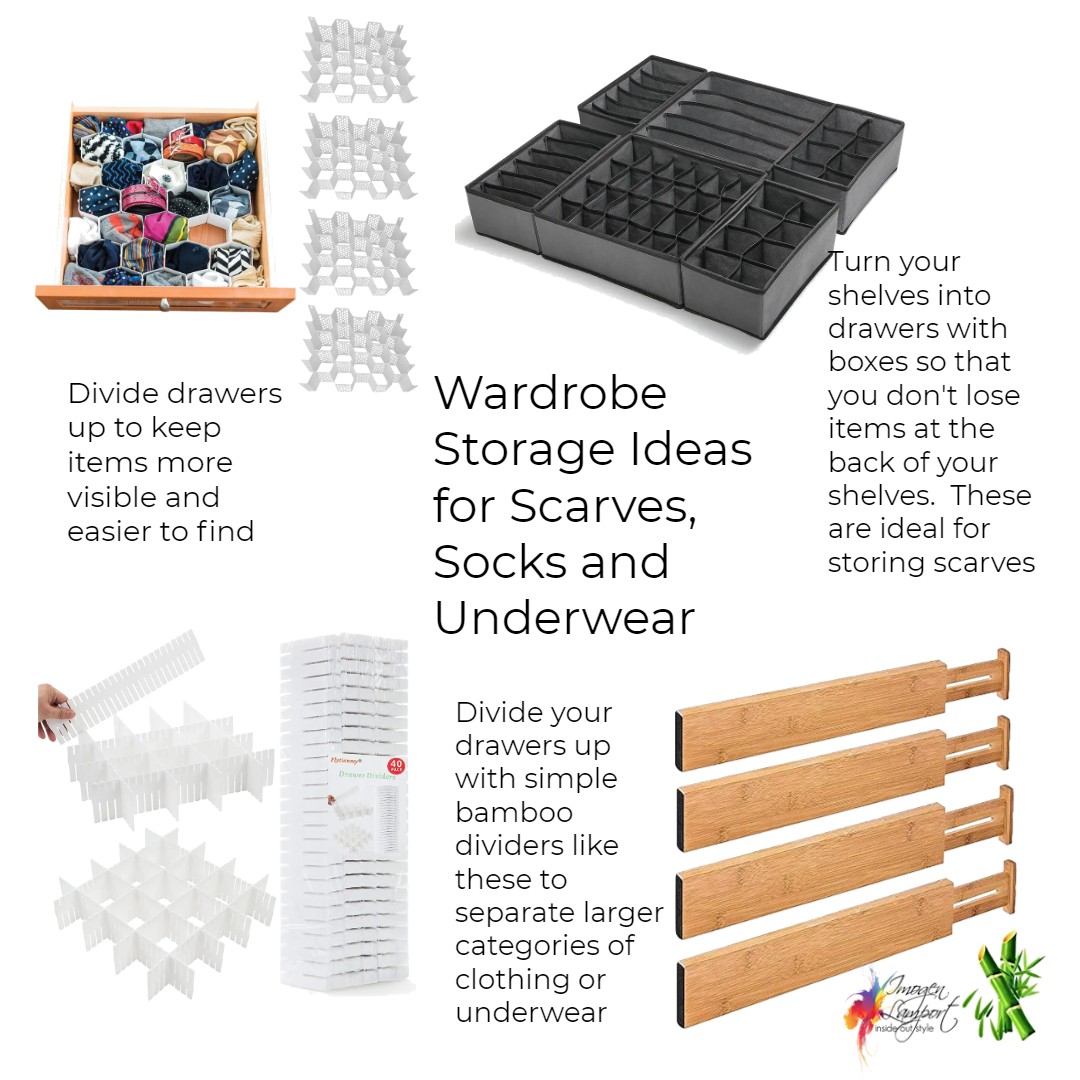The image is an advertisement showcasing various wardrobe storage solutions, set against a white background. Central to the image is the prominent text, "Wardrobe storage ideas for scarves, socks, and underwear." On the left side, there is a picture of a drawer with dividers installed, highlighting the use of hexagonal storage compartments and bamboo dividers. The associated text emphasizes, "Divide drawers up to keep items more visible and easier to find." On the right, another section features a dark gray tray with cut-out sections for organizing smaller items. Above it, the text instructs, "Turn your shelves into drawers with boxes so that you don't lose items at the back of your shelves." Below, on the bottom left, there are white storage containers, while on the bottom right, wooden dividers with a similar function are seen. The text on the right also reads, "Divide your drawers up with simple bamboo dividers like these to separate larger categories of clothing or underwear." The advertisement is visually framed with a green logo featuring bamboo stalks in the lower right corner, adding a touch of nature-inspired design.